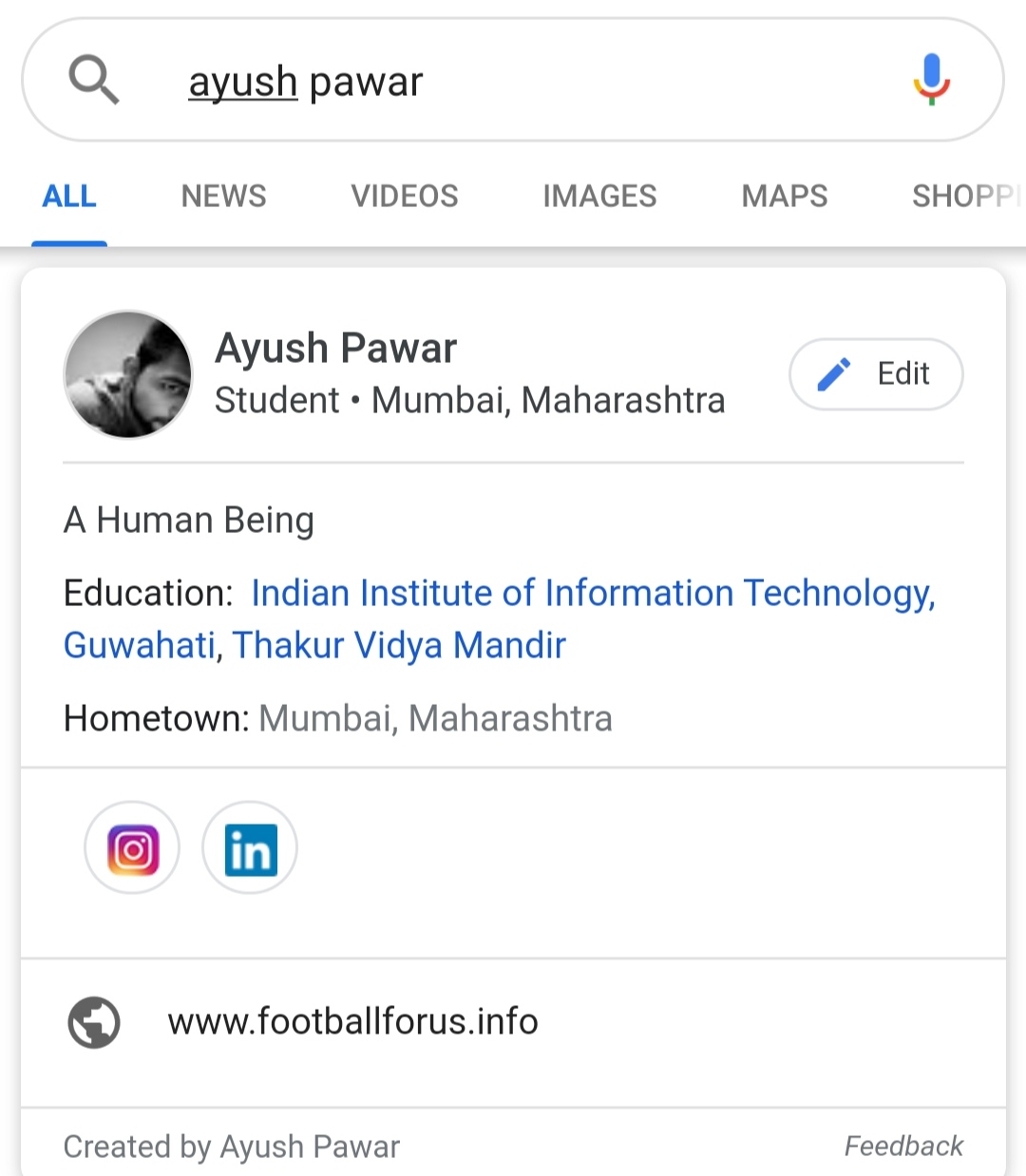The image displays a computer screen where someone has entered a search query for "AYUSH PAWAR" in an online search bar. The search bar also features a microphone icon, indicating the option for voice search. The user has selected the 'All' category from the search options, which include News, Videos, Images, Maps, and Shopping.

The search results bring up a profile for Ayush Pawar, identifying him as a student from Mumbai, Maharashtra. The profile picture is a black and white image of a young man, showing only half of his face as he leans downward. The profile includes an option to edit details, symbolized by a pencil icon.

The educational background listed states that Ayush Pawar attended the Indian Institute of Information Technology in Guwahati and Thakur Vidya Mandir. His hometown is noted as Mumbai, Maharashtra. Additionally, he appears to have an Instagram account and is also associated with another unspecified platform, represented by the abbreviation "NIN" on the profile.

A black and white picture of a globe and a blue box link to a website www.footballforus.info, attributed to Ayush Pawar.